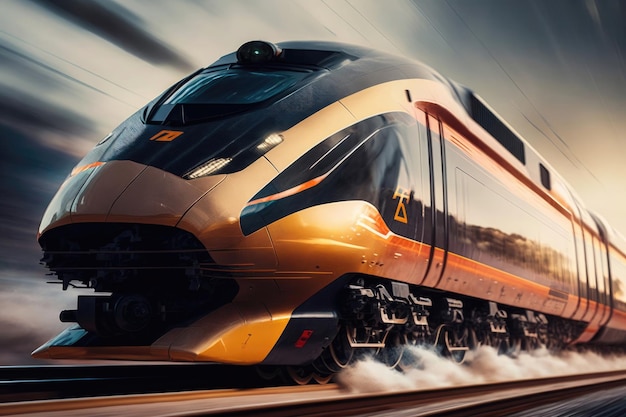This image depicts a highly modern, futuristic train, either digitally created or AI-generated, with a sleek and aerodynamic design. The train, predominantly gold and black with distinctive copper lines running along its side and top, features a large grill opening at the front and possibly a wing-like structure under its front bumper. The train is positioned on the tracks, clearly in motion, as indicated by the blur in the silver-ish background and steam or smoke emanating from its wheels. The train’s mirrored surface reflects the surrounding scenery, including trees, enhancing its dynamic appearance as it heads towards the left. There is no discernible text or signage on the train.